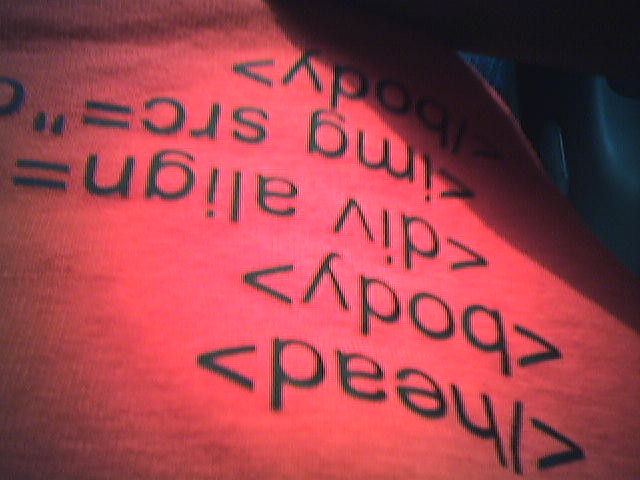In this intriguing, slightly surreal image, a red cloth is prominently featured, adorned with printed code—a curious choice of medium for such text. The photograph is taken upside down, capturing the cloth from bottom to top. Each line of code is encased in triangular brackets, sequentially reading: `<head>`, `<body>`, `<div align=...>`, `<img src=...>`, and then closing with `</body>`. Adding to the enigmatic scene, a crumpled blue fabric occupies the top right corner of the frame, creating a textured contrast against the smooth, code-printed red cloth. The unexpected juxtaposition of coding—typically confined to digital screens—printed on textile infuses the image with a sense of mystique and unconventional artistry.